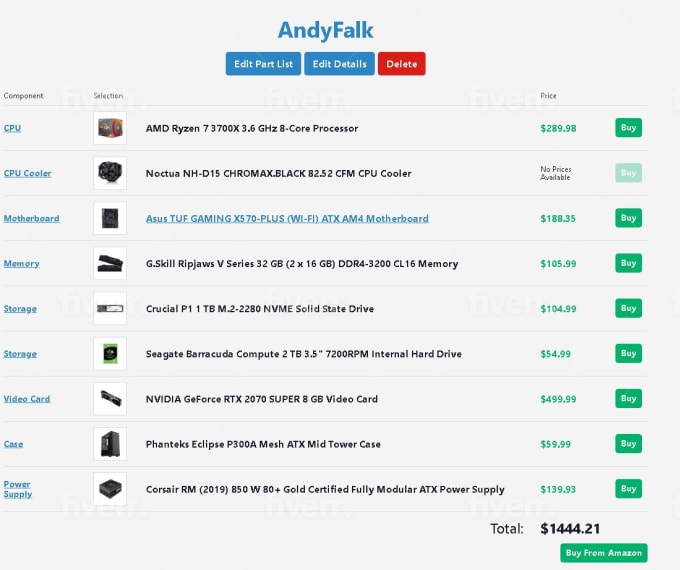The image displays a detailed web page from a site called "Antifock," which appears to specialize in computer hardware. The website's name "Antifock" is prominently highlighted in blue at the top. Beneath the site name, there is a blue button labeled "Edit Part List," enabling users to modify or delete parts from their list.

The page is organized into three columns: Component, Selection, and Price. The first component listed is the CPU, labeled as an AMD Ryzen 3.6 GHz 8-core Processor, priced at $289.98 in green, with an adjacent green "Buy" button. Following this is a CPU Cooler, specifically the Noctua NH-D15 Chromax Black, which currently has a "No price available" status.

Next on the list is the motherboard: an Asus TUF Gaming X570-Plus with Wi-Fi capabilities, available for $188.35, accompanied by a "Buy" button. The memory is specified as a G.Skill Ripjaws V-Series, priced at $105.99. Storage options include a solid-state drive (1TB Seagate Barracuda) for $104.99 and an Intel hard drive for $54.99. For graphics, the Neptiva GeForce video card is listed at $499.99.

Additionally, the case is a Phanteks Eclipse mid-tower available for $59.99. Powering the setup is a Gold Certified Fully Modular Power Supply listed at $139.93. The total cost for all selected items is $1,444.21, with a button beneath this total indicating the option to purchase all items directly from Amazon.